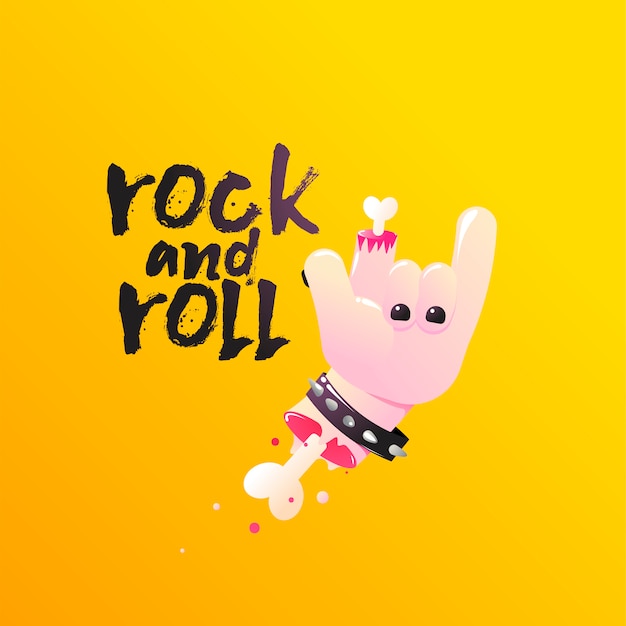The animated image features a detailed, graphic depiction of a left human palm making the rock and roll symbol, against a solid yellow background that gradates from a darker orange on the left to a brighter yellow on the right. In the middle, to the left of the hand, the words "rock and roll" are written in lowercase, black letters. The hand, with the palm facing front, has the thumb and pinky finger extended upwards, while the middle and ring fingers are down, showcasing black nail polish. Notably, the tip of the ring finger is sliced off, revealing a protruding bone with blood dripping from the wound. The bone resembles a stem with a heart on the end in its style. Additionally, the wrist is also severed, exposing a larger bone and drops of blood, with a purple spiky wristband around it. To the left of the palm, there's an element which includes a rock and a row, adding extra detail to the vivid and gruesome illustration.